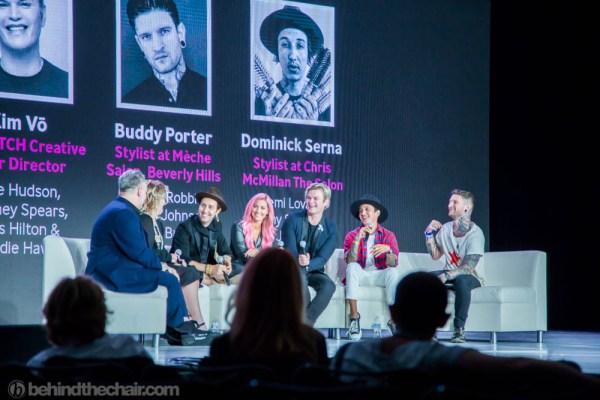This photograph captures a lively panel discussion on stage, featuring seven individuals, a mix of men and women, all dressed well and seated on white couches and chairs. They appear to be of varying ages, but share commonality in their engaged and friendly demeanor. Among the panelists, there's a man in a suit, a woman in a black dress, another man in a suit and a hat, a woman with pink hair, a man in a black hat, pink shirt, and white pants, and another man in a white shirt, pants, and covered in tattoos.

Behind the panelists is a large projector screen displaying black-and-white photographs of some of the panelists, with their names clearly visible in white text. Notably, the names "Dominic Serena" and "Buddy Porter" appear on the screen, followed by their titles, "Stylist at Chris McMillan the Salon" and "Stylist at Mecca Salon Beverly Hills," respectively, written in purple text. Additional text descriptions are present but partially obscured by the people seated on stage. 

In the foreground at the bottom of the image, you can see the back of the heads of audience members, hinting at a studio or conference setting. The overall atmosphere is warm and jovial, suggesting that both the panelists and the audience are enjoying the presentation.